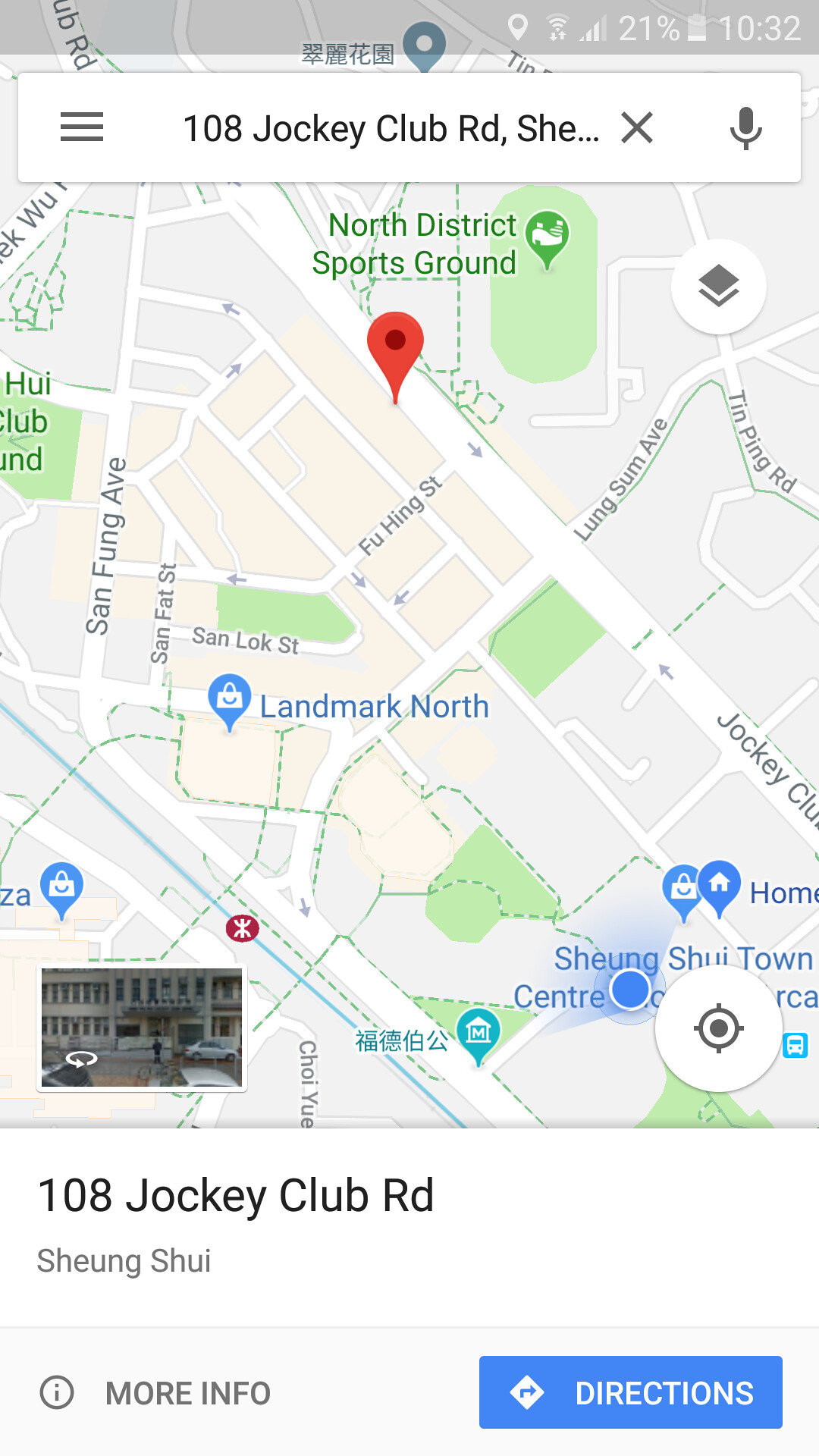The image is a screenshot from a cell phone displaying the Google Maps app. Prominently featured in the center is a map with a large red pin marking the location at 108 Jockey Club Road. The map background is light gray with white roads and green areas indicating grassland. Various roadways and landmarks such as Landmark North and Shengshu Town are clearly labeled. At the top, the address 108 Jockey Club Road is displayed, along with the status bar showing Wi-Fi signal strength, 21% battery life, and the time, which reads 10:32. Notably, in the bottom left corner, there's a small live street view photo of a building with a car parked in front of it, available for street view access. Below the map, the address is reiterated as 108 Jockey Club Road, Shengshui, accompanied by a banner for "More Info" and a clickable blue bar for directions.